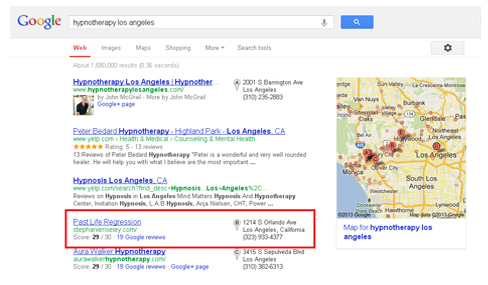This is a detailed, cropped screenshot of the Google desktop web search interface. At the top of the screen, there is a gray banner featuring the Google logo positioned on the top left. Centered within the banner is a search bar with the query "hypnotherapy Los Angeles" typed in lowercase letters. To the right inside the search bar, there is a microphone icon, and on the far right, outside the search bar, there is a blue square button with a white magnifying glass icon indicating the search function.

Below the gray banner, the body of the web page is displayed with a white background. On the right side of the web page, an embedded Google Maps image is visible. Directly below the map image, the text "map for hypnotherapy Los Angeles" appears in bold, blue font. To the right of the map, there is a list of search results. One specific listing towards the bottom of this list is highlighted by a red box, which has been edited into the photo to emphasize the business named "Past Life Regression."